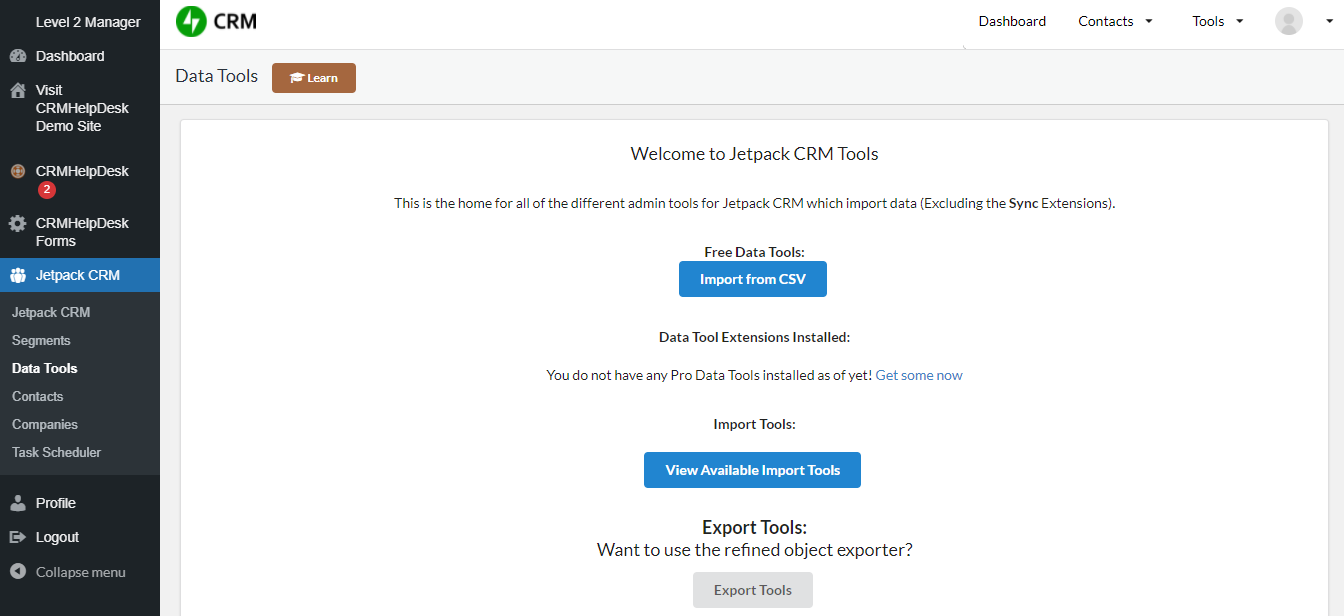**Caption:**

The image is a detailed screenshot of a desktop computer displaying the Jetpack CRM interface. 

**Left Menu Bar:**
- The menu bar is situated on the left side, characterized by a dark gray background and white text.
- The top section reads "Level 2 Manager".
- Various icons and options follow:
  - Dashboard
  - Visit CRM Help Desk Demo Site
  - CRM Help Desk (with a red notification bubble showing the number "2")
  - CRM Help Desk Forms
  - Jetpack CRM (displayed inside a blue box with a white logo)
  - Jetpack CRM Segments (in gray lettering)
  - Data Tools (in white lettering)
  - Contacts, Companies, and Task Scheduler (all in gray lettering)
  - At the bottom of the menu, there are options for Profile, Logout, and Collapse Menu.

**Right Menu Bar:**
- This appears to be narrower, with a white background and green CRM logo at the top.
- Menu items include Dashboard, Contacts, Tools, and the User Icon.
- Below these options is a gray bar labeled Data Tools, followed by a brown box with white lettering that says Learn.

**Main Content Area:**
- The main section of the page has a white background with the header "Welcome to Jetpack CRM Tools" in black letters.
- It highlights that this section is the home for various admin tools within Jetpack CRM such as data imports (excluding sync extensions) and free data tools.
- A prominent blue button labeled "Import from CSV" is visible for initiating data imports.
- The interface indicates that no pro data tools are installed by default, with a call to action in blue text "Get Some Now".
- Further options include Import Tools and another blue button labeled "View Available Import Tools".
- Bold black text reads "Want to use the Refined Object Exporter?"
- At the bottom is a gray box with "Export Tools" written in black lettering.

The entire interface is structured to provide a comprehensive overview of the functionalities and navigation within the Jetpack CRM system, aiding users in managing their customer relationship tasks effectively.